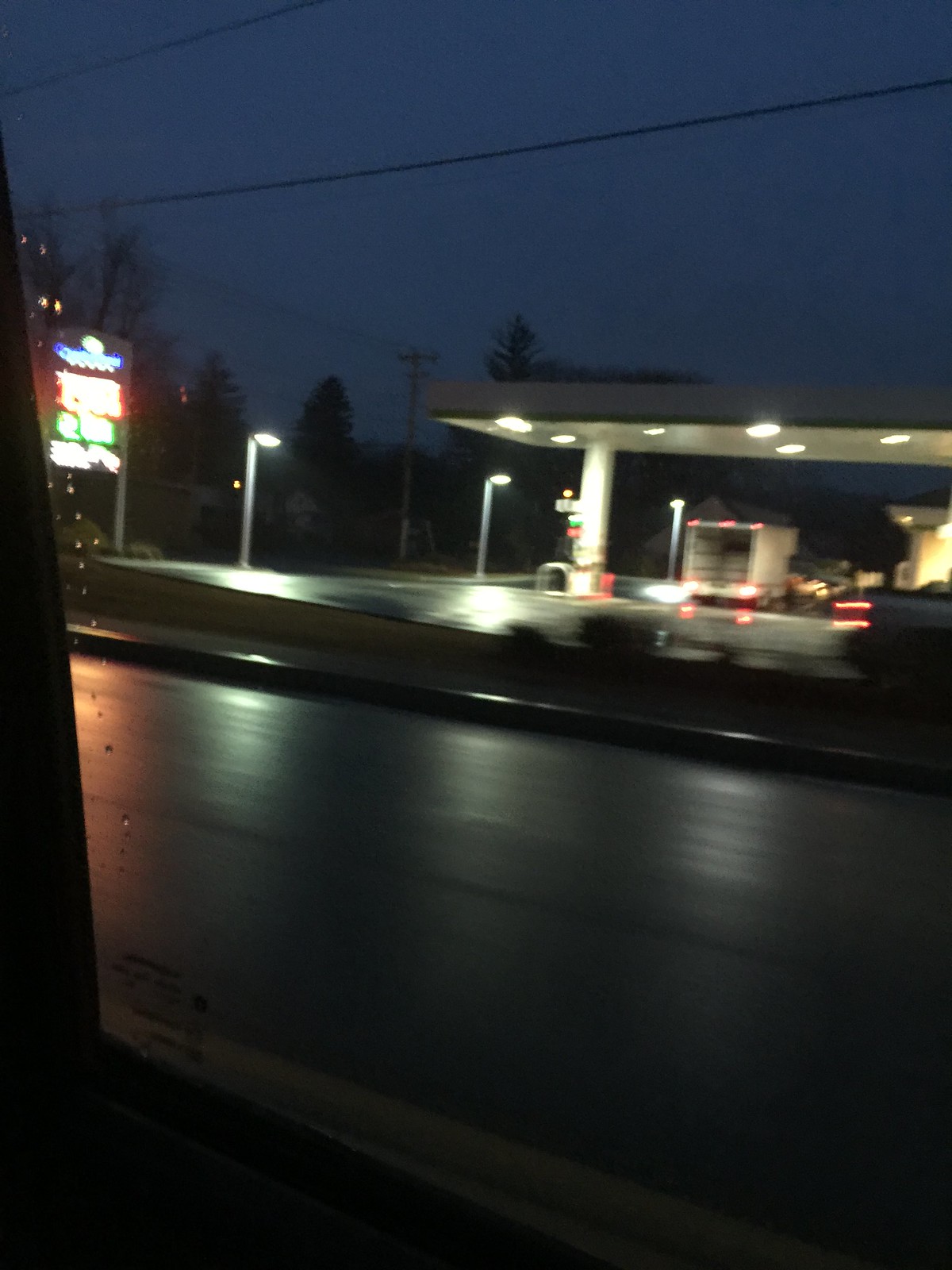The image captures a nighttime scene viewed through a window, with the left and bottom window frames visible in black. In the foreground, there's a gray road that appears wet, suggested by white light reflections forming three distinct patterns, along with a reddish-orange light to the left. Further back, a brightly lit, slightly blurry sign stands out, accompanied by two light posts to its right. A gas station, supported by a square-topped pillar, is prominently positioned in the middle ground. Dark green trees can be seen in the distance, and two telephone wires stretch across the scene. The top portion of the image showcases a serene blue night sky.